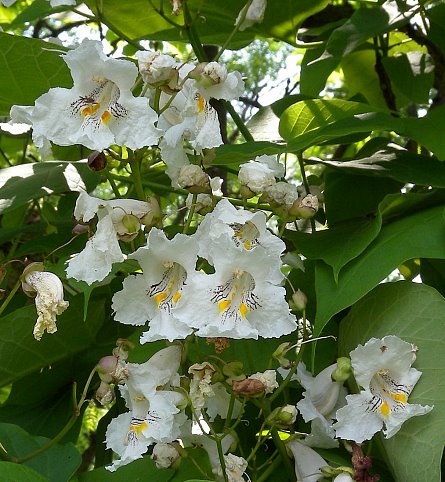This photograph captures a lush Northern Catawba plant in an outdoor setting, with a close-up view prominently featuring its delicate flowers. The plant’s verdant green leaves serve as a vibrant backdrop, contrasting sharply with the predominantly white, ruffled petals of the flowers. Each bloom is intricately detailed with yellow markings and delicate streaks of black or purple at the center. Sunlight filters through the foliage, illuminating the tender and somewhat delicate flowers, some of which are in full bloom, while others show signs of withering. The blue sky peeks through the upper part of the image, adding a natural serenity to the scene. Overall, the photograph highlights the plant's natural beauty, texture, and the gentle transition of its blooms.